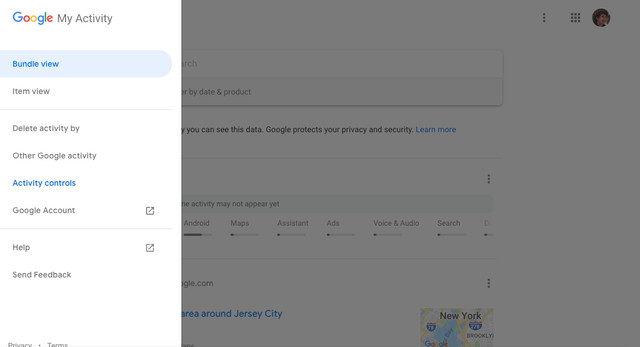The image is a screenshot of a Google My Activity page. In the upper left corner, the "Google" logo and "My Activity" text are clearly visible. Beneath the "Google My Activity" header, the user has selected the "Bundle View" option, as indicated by its highlighted state. Additionally, the "Activity Controls" in the same row is marked in blue, suggesting it is another interactive element.

To the right of this section, there is a large, slightly rectangular gray box that appears to be a cropped portion of another screen. In the upper left corner of this gray box, there is a small circular profile picture of a light-skinned individual with dark hair. Below the profile picture, the text "Google protects your privacy and security" is partially visible.

Within the gray box, several labeled bars can be discerned, including those for "Android," "Maps," "Assistant," "Ads," "Voice," and "Audio Search." At the bottom left of this section, a link or label in blue text reads "Around Jersey City."

Towards the bottom center-right of the image, partially peeking into the frame, is the top portion of a map. The map features prominent labels including "New York" at the top and "Brooklyn." This map fragment also displays bodies of water and highways, adding geographical context to the visible regions.